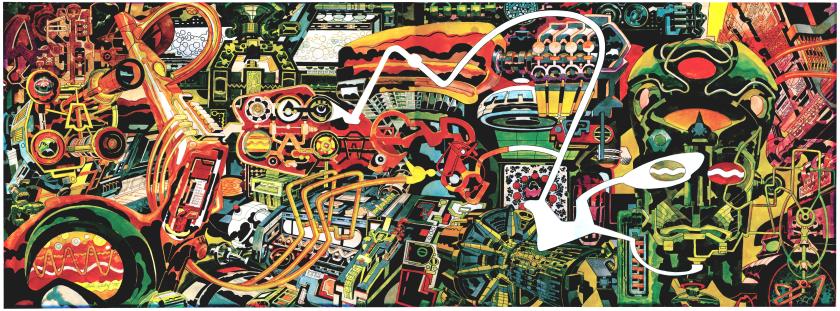This intricate and colorful rectangular artwork, reminiscent of a futuristic town or the inside of a highly detailed machine, bursts with vibrant hues including white, orange, red, green, blue, teal, black, and yellow. The drawing, almost in a playful, graffiti-like style, features an array of components tied to motors and electronics, interconnected by a complex network of wires, tubes, and gears. A prominent white wire arcs across the image, breaking up the intense color palette. On the bottom left, a green circular shape filled with orange wavy lines stands out against a red background, with another white wavy line behind it. Above this, a square-like object adorned with circles at each corner adds to the densely packed visual narrative. There is barely any negative space, as every inch is filled with imaginative, machine-like structures, making the scene appear almost alive with motion and energy.